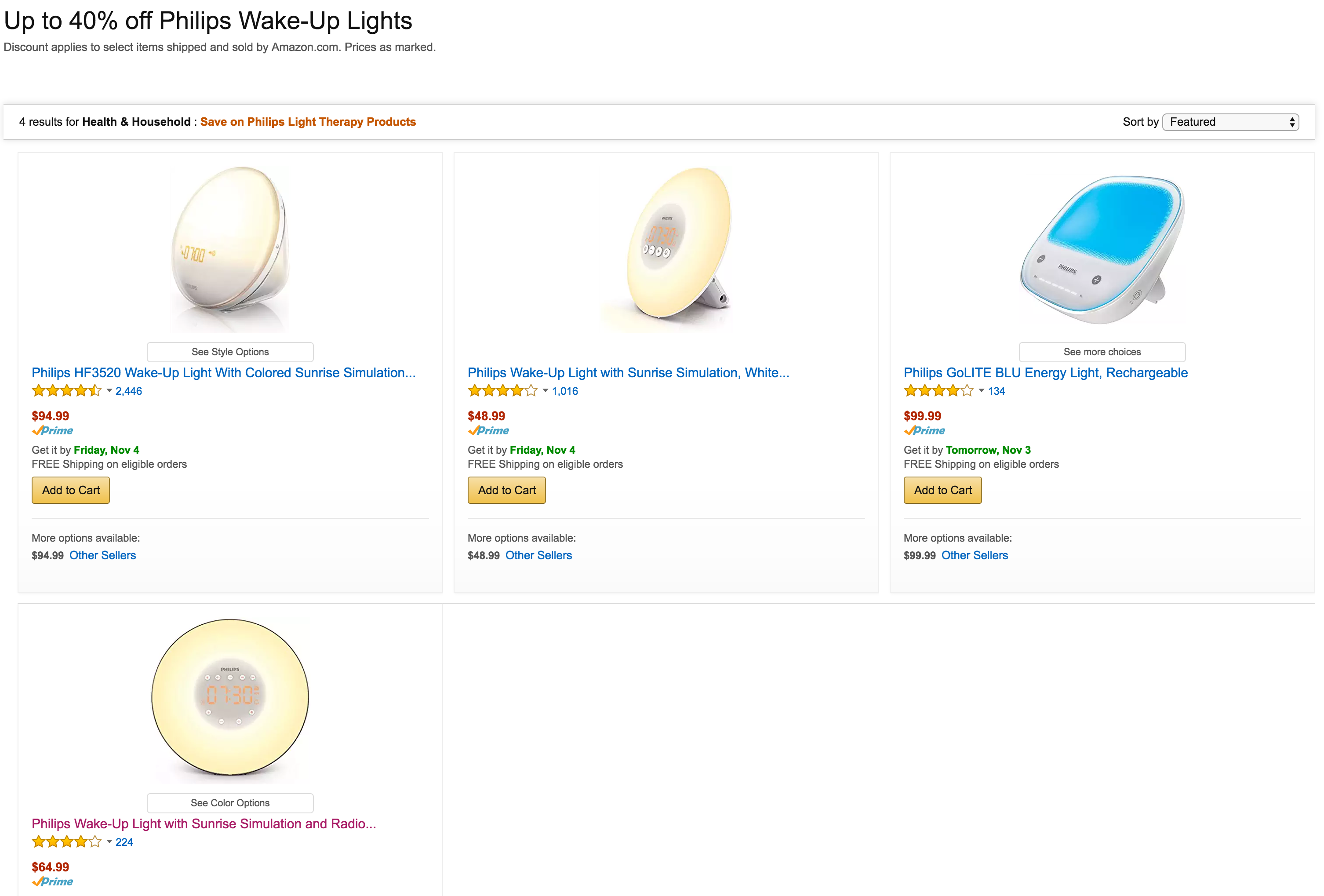This image portrays an online shopping page dedicated to Philips Wake Up Lights with a promotional banner at the top announcing "Up to 40% off Philips Wake Up Lights." The page specifies that the discount is applicable to select items shipped and sold by Amazon.com, with prices already marked down. Underneath the header, it is stated that there are 4 results for the "Health and Household" category, encouraging shoppers to save on Philips Light Therapy products. The page displays four product options:
1. **Philips HF3520 Wake Up Light with Colored Sunrise Simulation**:
   - **Rating**: 4.5 stars based on 2,446 reviews
   - **Price**: $94.99
   - **Shipping**: Eligible for Amazon Prime with free shipping and delivery by Friday, November 4th
   - **Additional**: "See style options" link and an "Add to Cart" button

2. **Philips Wake Up Light with Sunrise Simulation in White**:
   - **Rating**: 4 stars based on 1,016 reviews
   - **Price**: $48.99
   - **Shipping**: Eligible for Amazon Prime with free shipping and delivery by Friday, November 4th

3. **Philips Go Light Blue Energy Light Rechargeable**:
   - **Rating**: 4 stars based on 134 reviews
   - **Price**: $99.99
   - **Shipping**: Available through Amazon Prime
   - **Additional**: Features a blue color with a silver body

4. **Philips Wake Up Light with Sunrise Simulation and Radio**:
   - **Rating**: 4 stars based on 224 reviews
   - **Price**: $64.99
   - **Additional Features**: Includes a radio, displays the time (7:30 AM) in orange on a central Philips screen, and emits a bright light

The page predominantly features a white background with product images showcased alongside their respective details.